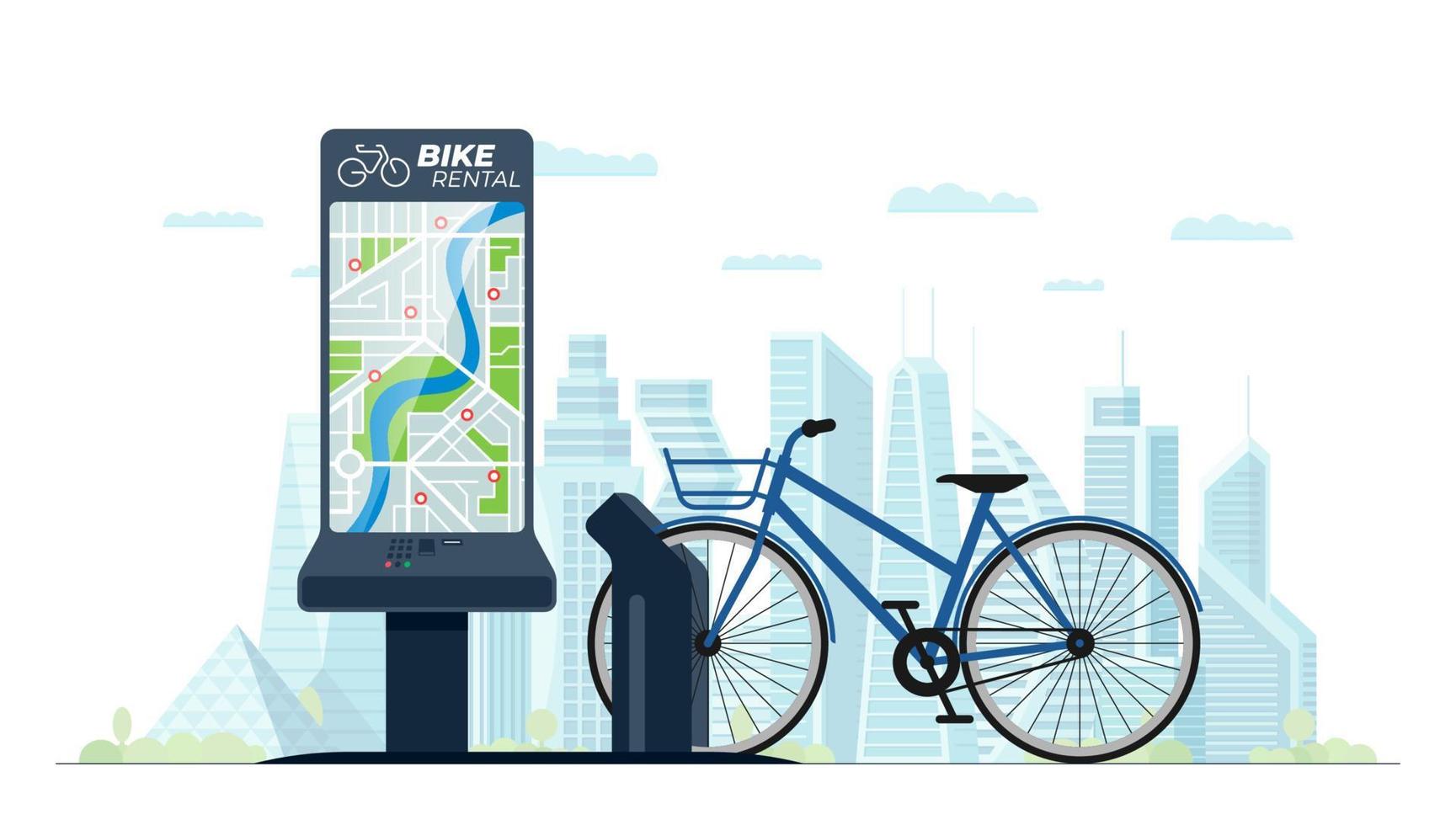The image depicts a detailed computer illustration of a bicycle rental station typically found in large cities, highlighting the ease of renting and using bikes for urban transportation. The station features a blue bike with a basket securely locked into its rack. A kiosk with a card reader is central to the image, complete with a screen displaying a map adorned with red dots, indicating various bike rental locations throughout the city. The backdrop features a cartoon-like silhouette of a cityscape, complete with towering skyscrapers, clouds, and a touch of grass in the lower corner, symbolizing urban green spaces. This illustration aims to promote the convenience of a bike-sharing program, showcasing how users can effortlessly rent a bike, use it to navigate the city, and return it to any station. The presence of iconic buildings suggests this is a familiar service in major cities like Chicago, New York, and San Francisco, catering to both avid cyclists and casual users looking for efficient city travel options.